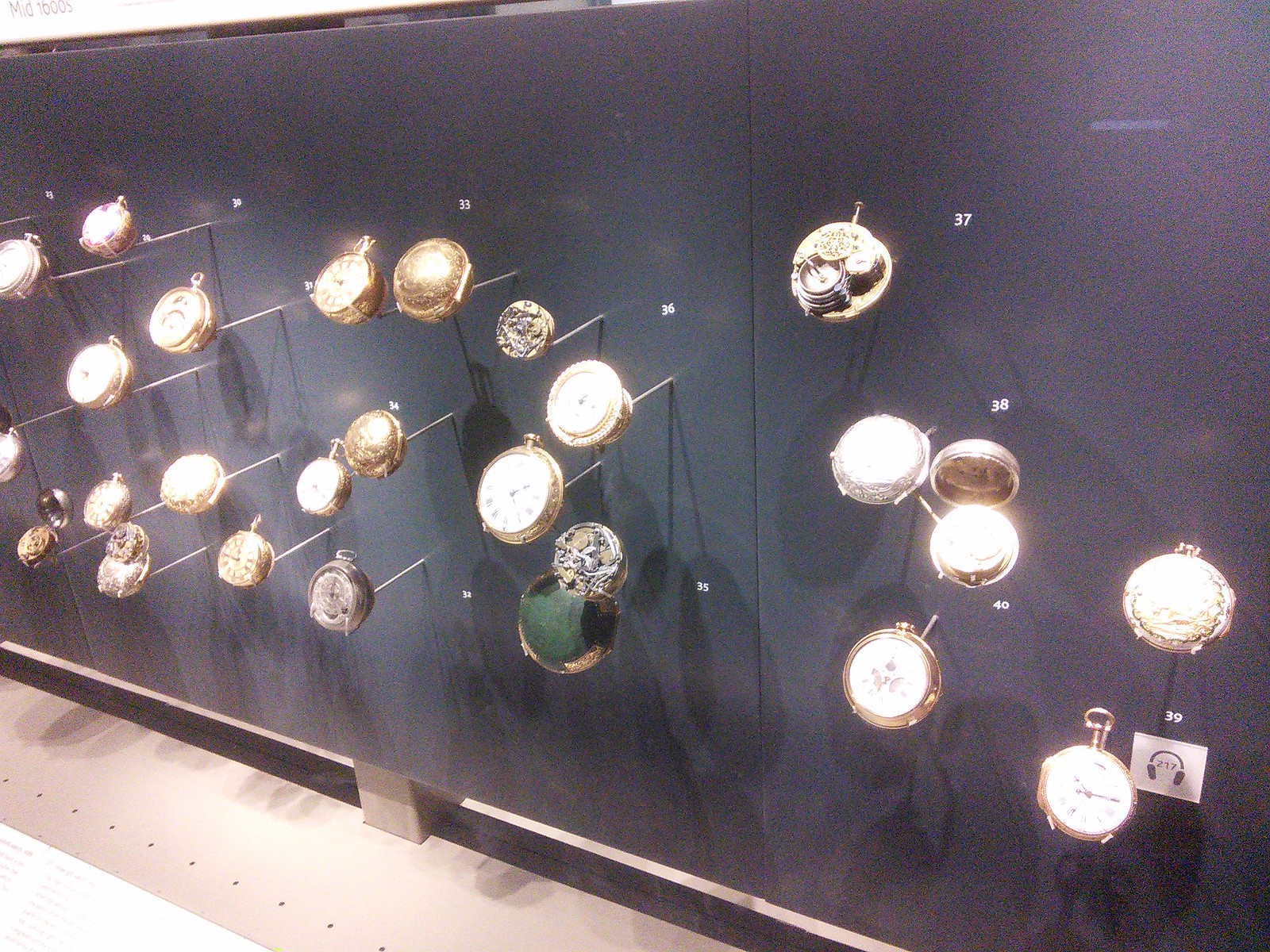The image shows a gray partition wall adorned with over a dozen various timepieces, resembling a collection of pocket watches or small clocks. These timepieces are attached to the wall by thin metal rods that protrude several inches, making them not flush with the wall. Each timepiece varies in shape, size, and ornateness, with many showing reflective, shiny surfaces that may obscure some details. The clock faces are accompanied by numbers on the wall, starting roughly around 28 or 29 up to 39, suggesting some form of numerical display backdrop. The floor beneath the wall is a mix of beige and white, providing a muted contrast to the metallic gleam of the predominantly gold and silver timepieces.